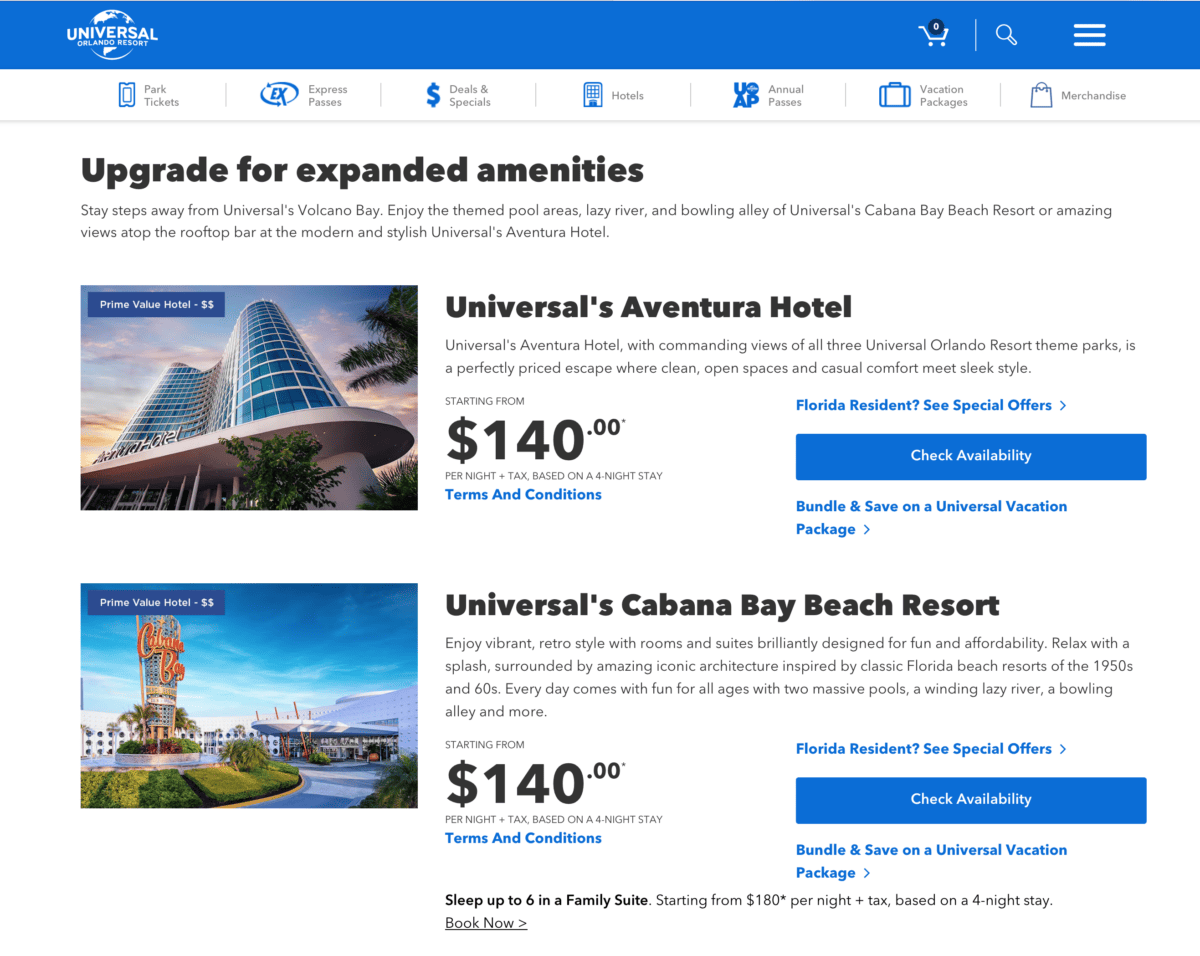The webpage from Universal Resorts, specifically showcasing Orlando Resorts, features a prominent blue navigation bar in the upper left-hand corner. An image of the resort can be seen within this bar, alongside an icon indicating items in the shopping cart, represented by a black circle with a number inside.

The options listed for purchase on the site include park tickets, express passes, special deals, hotel accommodations, packages, and merchandise. A highlighted section in bold black text emphasizes the opportunity to "upgrade for expanded amenities," encouraging visitors to stay just steps away from Universal's Volcano Bay. There's a promotional focus on the themed pool areas, Lazy River, and Bowling Alley at Universal's Cabana Bay Beach Resort, along with the modern amenities and scenic rooftop bar at Universal’s Adventure Hotel.

The page displays a striking ground-up image of one of the hotels, showcasing its very modern and sleek, round design. The hotel, identified as Universal's Adventure Hotel, offers rooms starting at $140 per night, with terms and conditions accessible via a blue link. A blue box provides options to explore special offers for Florida residents, check room availability, and more.

Just below, another featured section promotes Universal's Cabana Bay Beach Resort, also starting at $140 per night under similar terms and conditions. Both ads on the page promote the benefit of bundling for savings on vacation packages, mentioning the availability of family suites that accommodate up to six people, starting from $180 per night plus tax based on a four-night stay, with a "book now" option.